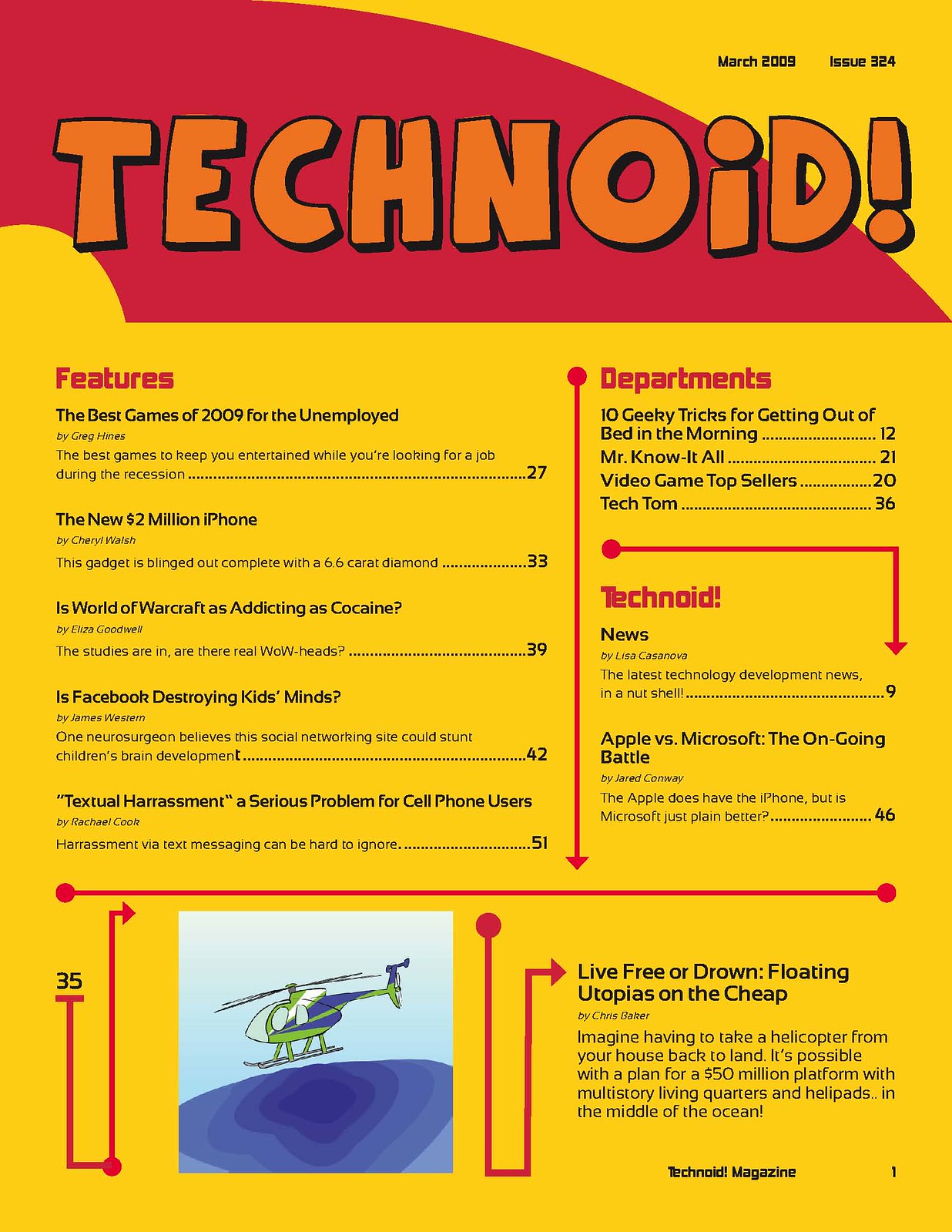This detailed descriptive caption incorporates shared and repeated information from both narrations, emphasizing commonalities and details:

This image appears to be a title page or placard from a technology magazine named "Technoid," featuring a mustard yellow background with some red accents. "Technoid" is prominently displayed in large orange font at the top, with a red area behind it for emphasis. The date "March 2009" and "issue 324" are indicated at the top in black text. The page provides an organized breakdown of features and departments within the magazine, including highlights such as "The Best Games of 2009" and "The New $2 Million iPhone." Specific articles listed include "The Best Games for the Unemployed" on page 27, "Is World of Warcraft as Addicting as Cocaine?" on page 39, and "Is Facebook Destroying Kids' Minds?" on page 42. At the bottom of the page, there is a drawing of a helicopter landing on water, with the caption "Live Free or Drown: Floating Utopia on the Cheap." This title page serves as a detailed guide to the magazine's contents, directing readers to various departments and features.